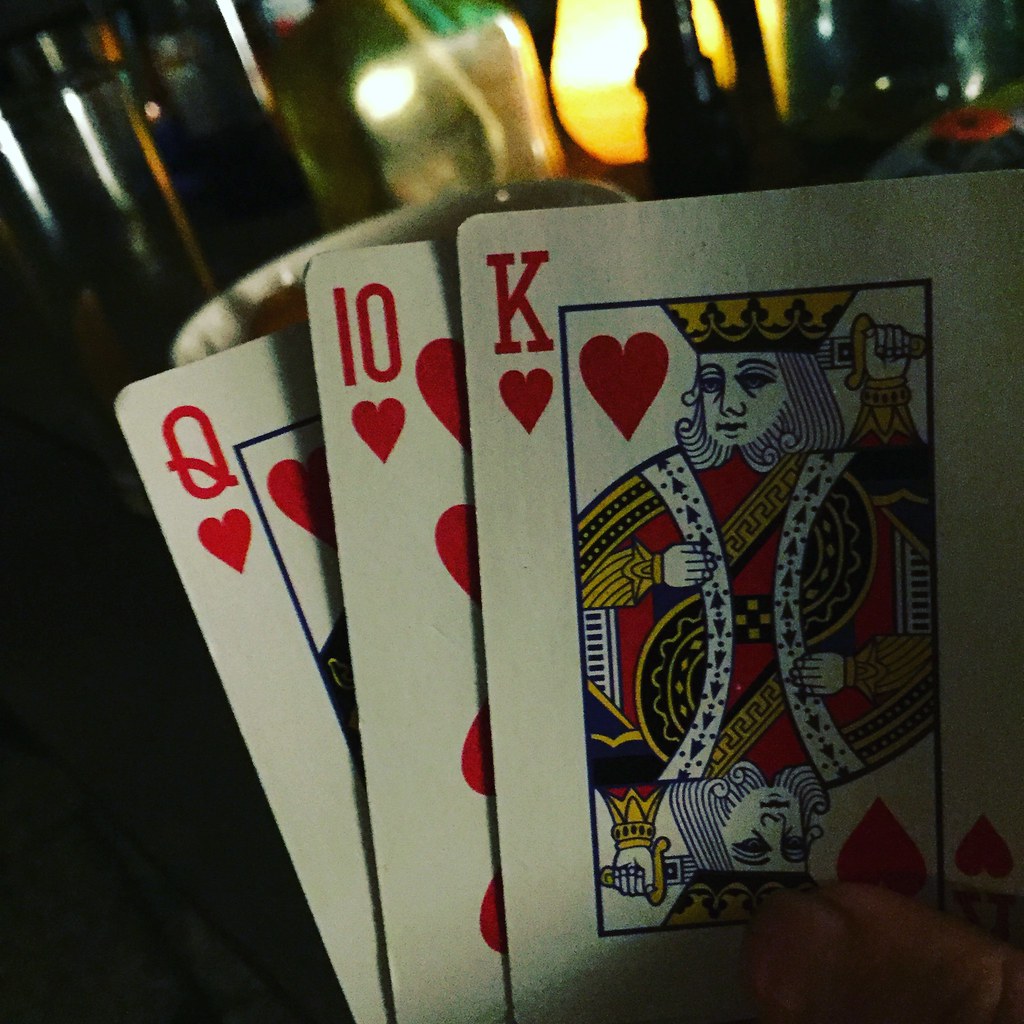In a dimly lit scene, a close-up focuses on a hand holding three playing cards – the Queen of Hearts, the Ten of Hearts, and the King of Hearts – displayed from left to right. Shadows dance on the King of Hearts, adding depth to the scene. The background is softly illuminated, possibly by a candle or a dim light source, creating a cozy, mysterious ambiance. A collection of what appears to be bottles sits on a table, with a clear glass containing a yellow star nestled among them. Just behind the cards, the white rim of a coffee cup is visible, partly obscured by the hand holding the cards. Flecks of light and shadow flicker throughout, enhancing the image's atmospheric quality.